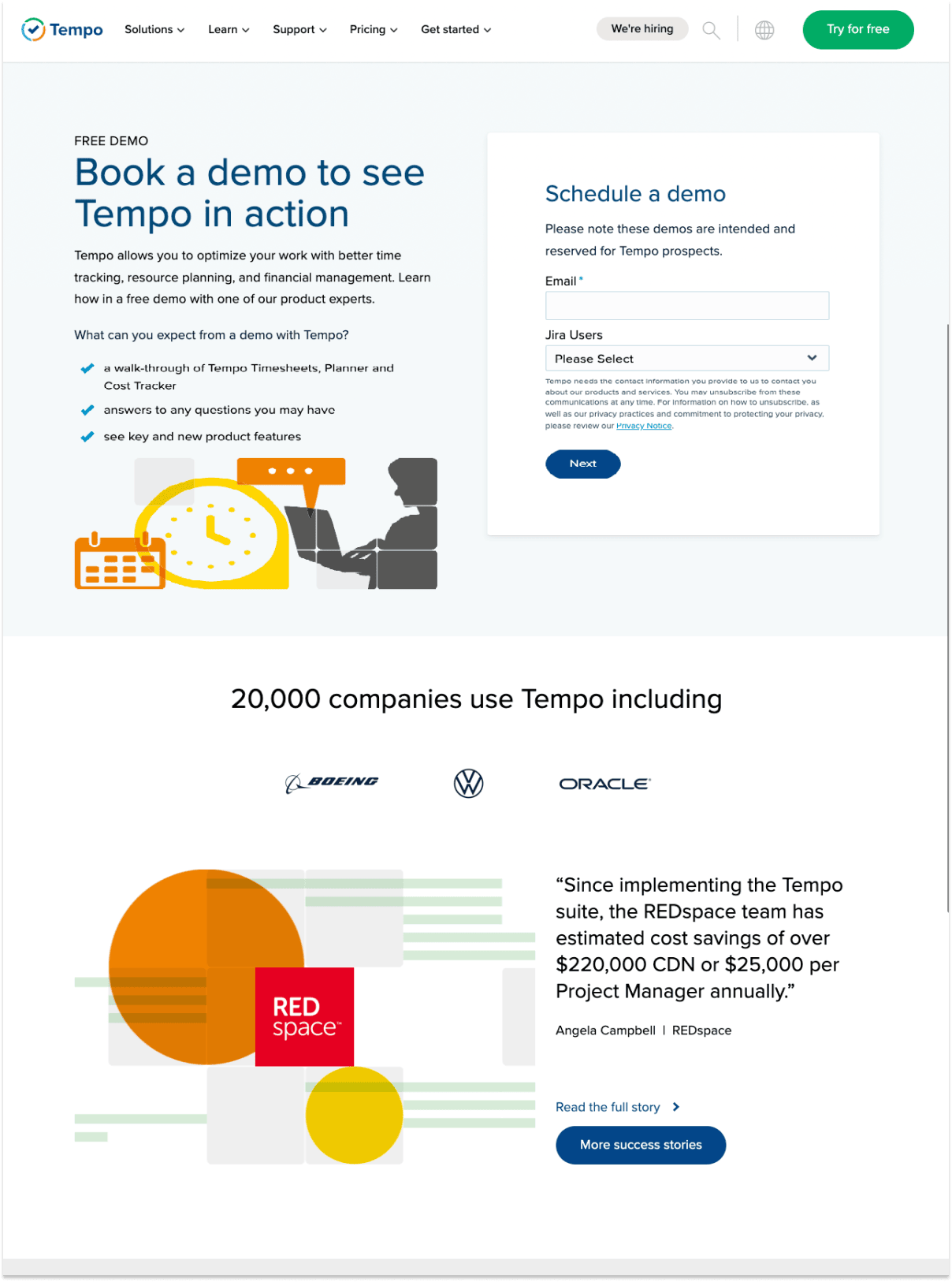This image is a screenshot from a website with a structured and colorful design.

The top portion features a white border, followed by a light blue section that extends halfway down the page, and then transitions into another white section at the bottom. 

At the very top, there is a multi-colored circle with a gradient: green at the top, yellow along the right side, and blue up the left side. Next to this circle is a blue checkmark, and the word "Tempo" written in blue text. 

Directly beneath that, in black text, are navigation options: "Solutions," "Learn," "Support," "Pricing," and "Get Started," each accompanied by a drop-down arrow. 

On the right side of the navigation bar, there is a green tab with "Try for Free" in white text. Adjacent to this tab, there is a circle with a grid pattern of three vertical lines intersecting with three horizontal lines, a small gray vertical line, and a search icon. Further right, there is a gray tab that says "Black, We're Hiring."

In the blue section below, the text on the left side reads "Free Demo." It continues with the tagline "Book a Demo to See Tempo in Action," followed by three lines of descriptive information and the header "What Can You Expect from Tempo," which features three blue checkmarks, each with accompanying text.

At the bottom of this section, there is a small orange calendar icon, a large yellow clock icon, and a shadow of a person holding a laptop on the right side. To the right, there is a tab that says "Schedule a Demo," with areas to input an email address and other details.

In the lower white section, the centered text proclaims, "20,000 companies use Tempo, including," followed by logos or names of companies such as Boeing, Volkswagen, and Oracle. 

On the right side of this section, there appears to be additional information, while on the left, there is a big orange circle. Below and to the right of this circle, there is a red square with "Red Space" written in white text, and beneath it, a smaller white circle.